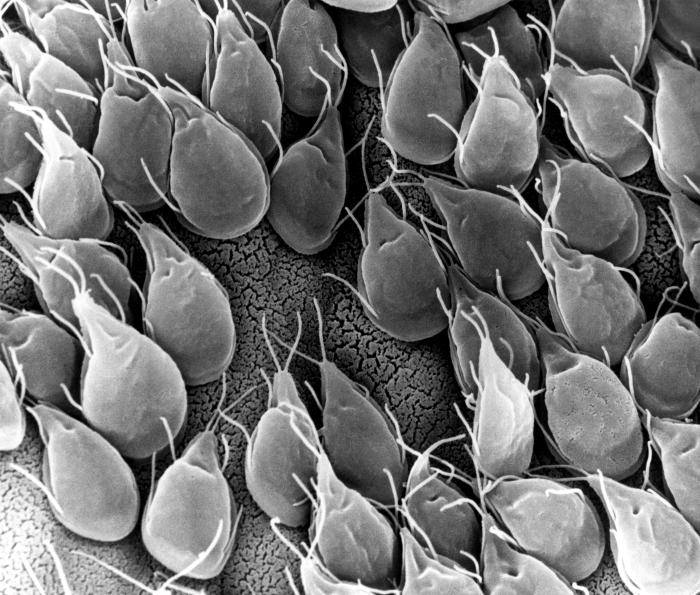The black and white image appears to be a highly magnified microscopic view of a surface densely populated by teardrop-shaped organisms. The organisms, which bear a resemblance to tiny insects or possibly scaled plants, come in various shades of gray and white, suggestive of a thermal imaging effect. These organisms have smooth, soft textures with some featuring legs or feelers extending from their tops, the lengths of which vary. The surface beneath them is cracked with dark squiggly lines, and the organisms almost entirely obscure it, especially in the top left and top right corners. In these areas, the concentration of organisms is so dense that the underlying surface is nearly invisible.